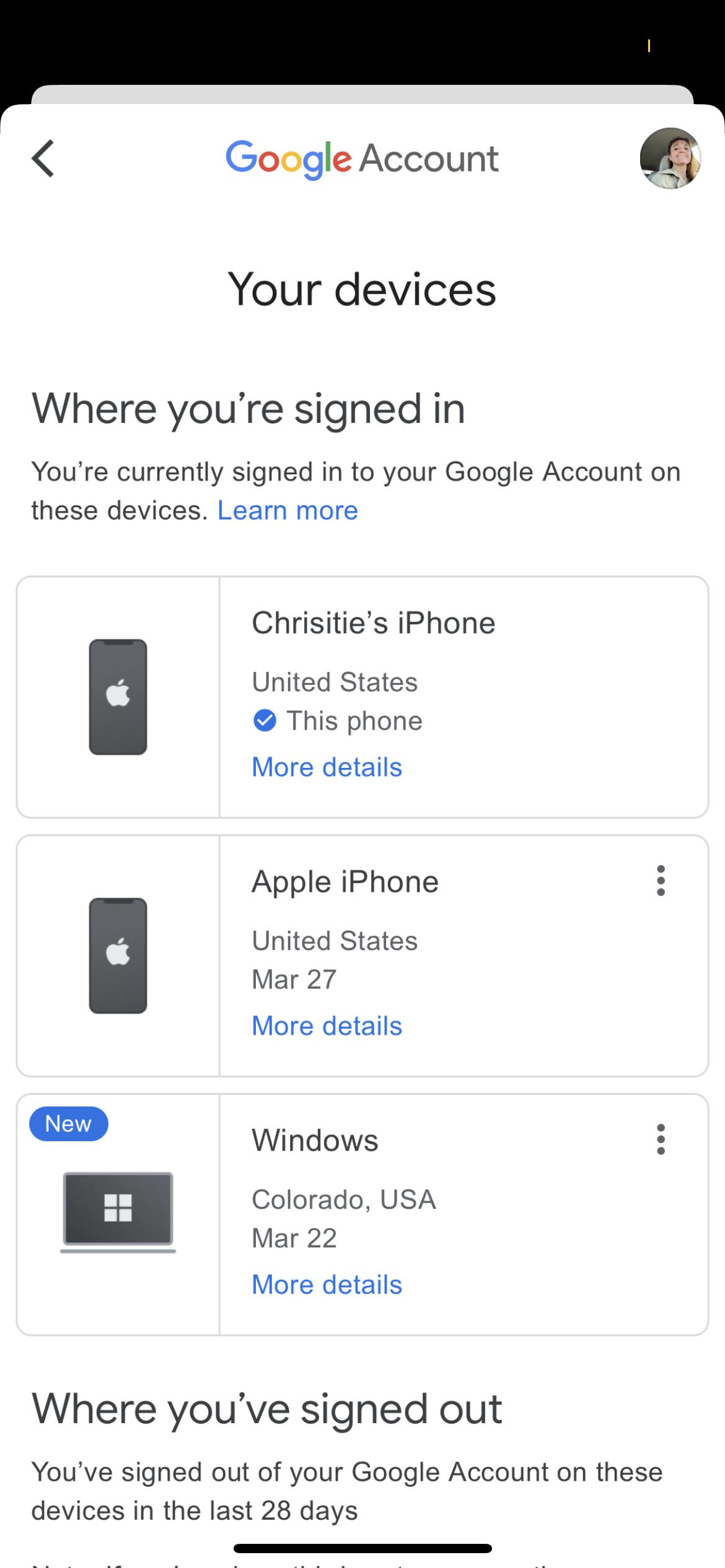This image is a cropped screenshot from a mobile device, displaying a mobile application interface. The top section of the screenshot is blacked out, possibly to hide specific details or notifications. Directly below the blacked-out area, the Google logo is prominently displayed with the word "Account" next to it. In the top right-hand corner, there is a circular profile picture of a woman. The main title of the window is "Your Devices," indicating the section where device activity is monitored.

The window lists three devices currently signed in with the Google account. The first device listed is "Christie's iPhone," located in the United States, which is the device from which this screenshot is taken. The second device is another iPhone, and the third is a Windows computer. Below the list of active devices is a section titled "Where you've signed out," which shows devices that the user has signed out from in the past 28 days. This section, however, has been cropped out and is not visible in the screenshot.